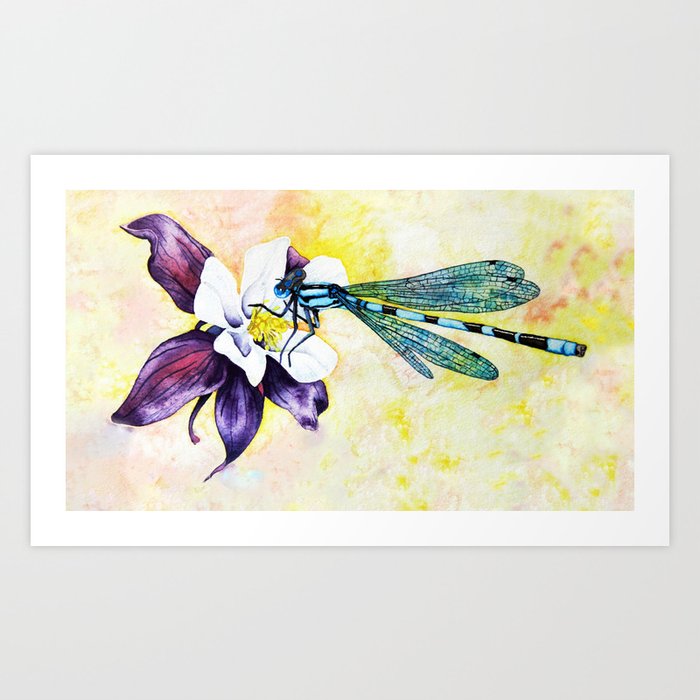The illustration depicts a blue dragonfly with black and white stripes perched on a flower. The artwork is framed by a thick white border. Within the scene, the dragonfly rests on one of the five rounded white petals that surround a central cluster of yellow sprigs. Below these white petals are long, pointed, shiny purple petals. The dragonfly, with its black and blue body and wings that reflect shades of blue and green, delicately interacts with the flower. The background of the painting features a soft, tie-dye-inspired blend of pastel colors, including pink, yellow, and white, creating a tranquil and ethereal backdrop. The painting is displayed on a wall, capturing the viewer's attention with its intricate details and harmonious color palette.